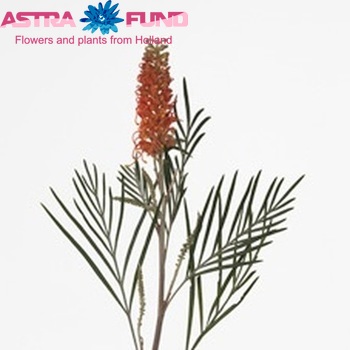This photograph appears to be designed either as an advertisement or as the front cover of a magazine issue. Dominating the top left corner of the image, the words "ASTRA Fund" are prominently displayed in a sleek, modern font, rendered in vibrant pink, capital letters. Positioned between "ASTRA" and "Fund" is an image of a delicate blue flower, adding a touch of elegance to the title. Beneath the main heading, a subtitle reads, "Flowers and Plants from Holland," offering insight into the content or theme.

Commanding the central focus of the photograph is a striking flower, likely belonging to the ASTRA variety. This single, tall cone flower stands proudly amidst lush green evergreen-like leaves. The flower itself boasts a light orange hue, exuding both simplicity and beauty. The background of the image is a pristine white, ensuring that the flower remains the sole focal point, undistracted by any additional elements. This minimalist composition highlights the natural allure of the plant, making it a compelling visual centerpiece.